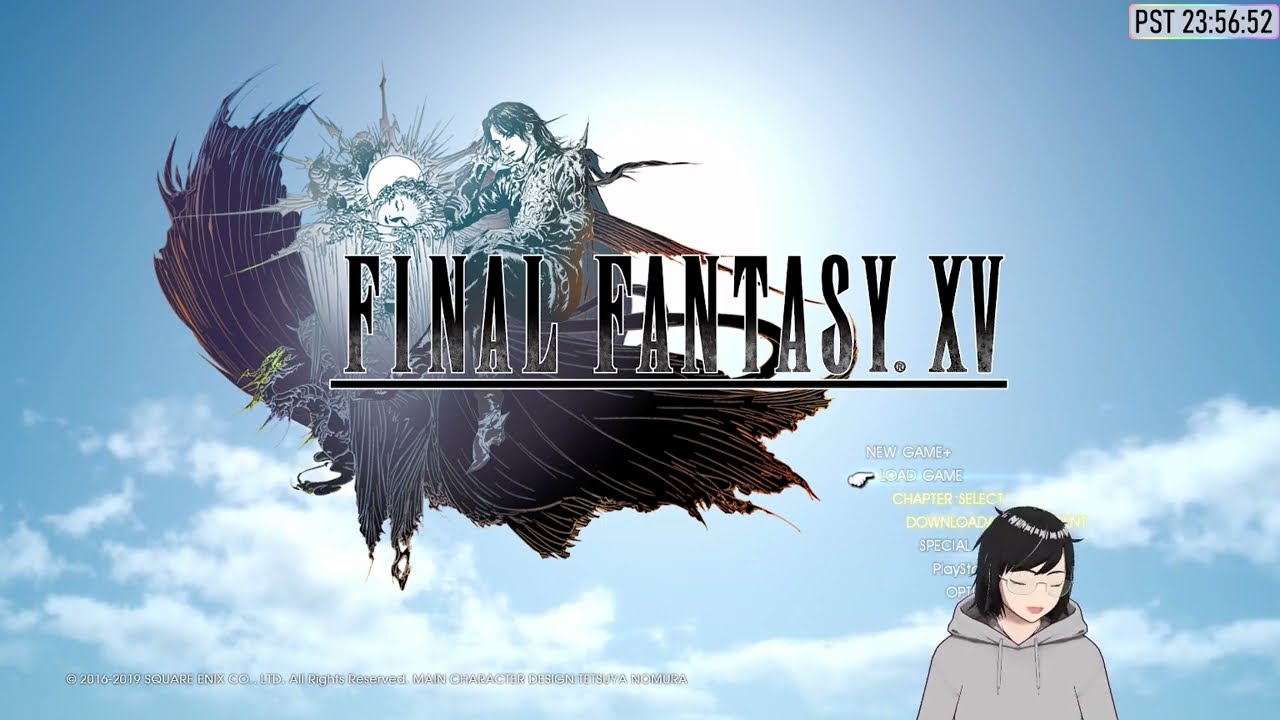The image depicts a highly detailed, stylized title screen for the video game, *Final Fantasy XV*. At the center, in bold black font with a black line underneath, is the game's title, "Final Fantasy XV". Below it are menu options that include "New Game", "Load Game", "Chapter Select", "Download", and "Special", all presented in different colors, with some options partially obscured by a character illustration. 

The lower right corner features a striking image of an Asian girl wearing a gray hoodie, short black hair, pink lips, and large round glasses. She is looking down with her eyes closed, her bangs curving to the left side of her face. Above and to the left, partially obscured by the title, are two women depicted in shades of black and gray. The first woman, with a cloak flowing behind her in hues of black, brown, light purple, and touches of orange, is seated on a dragon-like creature whose head is not visible, but its purple wings are noticeable. Beside her, another woman lies with her eyes shut, head resting on her hands. The backdrop features a serene blue sky with fluffy white clouds, enhancing the dreamlike quality of the scene.